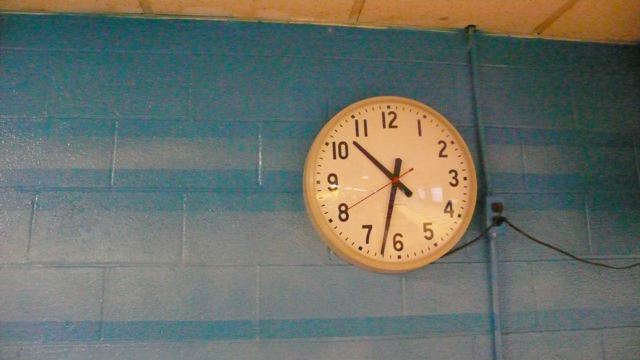The image showcases a large, classic classroom clock mounted high on a concrete wall. The clock features a beige face with a matching beige trim and has big, bold, black block numbers. The hour and minute hands are also black, while the second hand is a striking red. The wall behind the clock is adorned with horizontal stripes: a section of teal and blue at the top transitions into light blue downwards. The scene includes a white dropped ceiling and a visible conduit pipe protecting an electrical connection. A black cord extends from the clock to an electrical plug on the wall, suggesting the clock is plugged into the power source there.